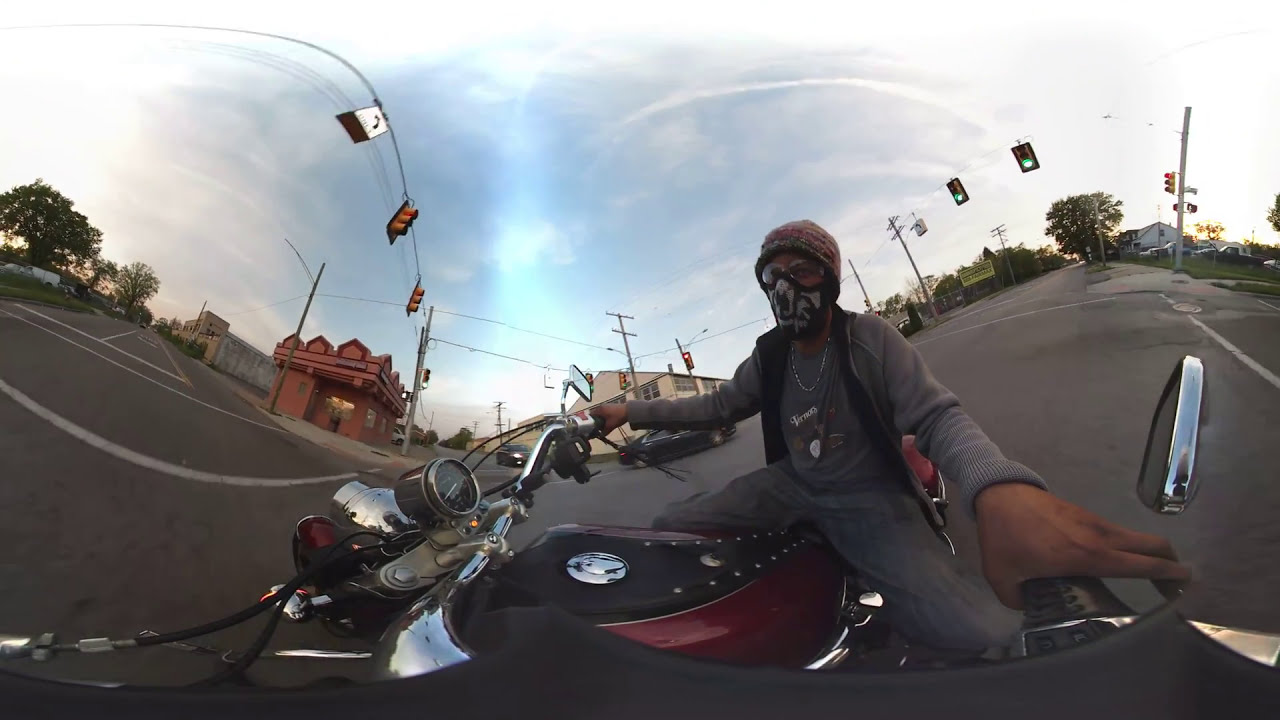In this detailed 360-degree panoramic photo, a male motorcyclist with dark skin is prominently featured at the center of the image, riding a large, deep burgundy-red motorcycle. The camera, positioned on one side of the bike's handle, captures a wide view of the scene. The biker is dressed in long gray pants and a long gray shirt, complemented by a beanie, goggles, and a unique face mask drawn to resemble a black and white mouth. The motorcycle is being ridden on a street paved with asphalt, through an intersection with a visible green traffic light over his shoulder, situating him in a city-like environment. Surrounding him is a mix of red and white buildings, trees, and bushes, with several streetlights scattered around. The sky above is mostly blue with some scattered clouds, indicating that it is a bright day. The entire frame is filled with colors such as gray, white, red, silver, black, green, and blue, contributing to the vivid depiction of the scene.